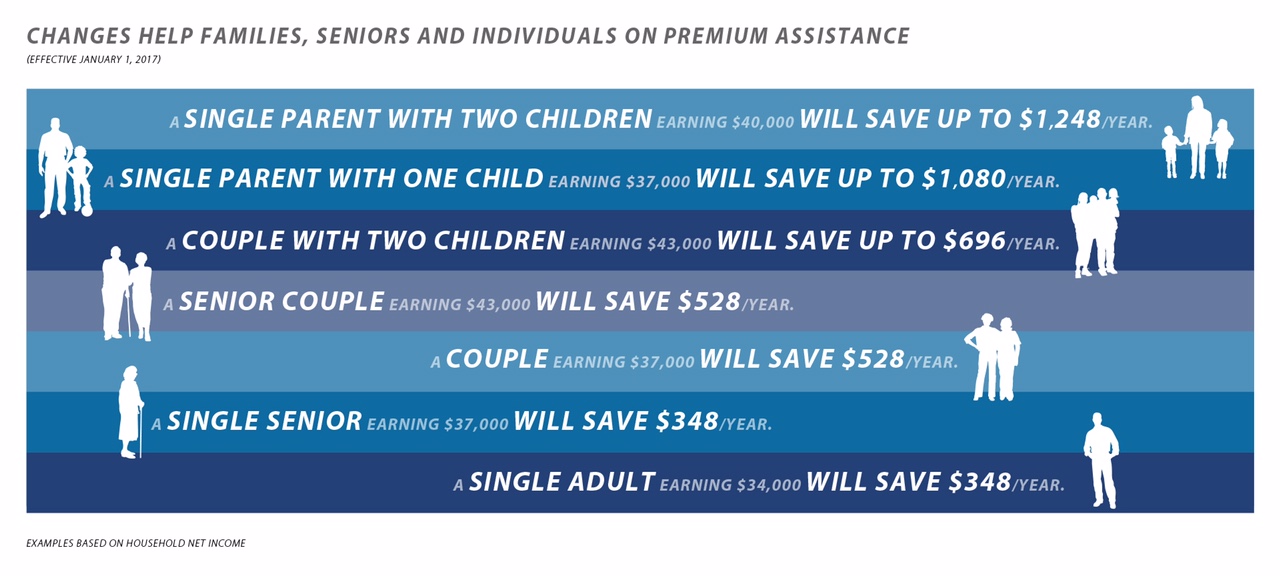The image is a detailed infographic presenting financial savings for different types of households due to changes in premium assistance effective January 1st, 2027. The top section, in gray text, reads, "Changes help families, seniors, and individuals on premium assistance effective January 1st, 2027." The infographic employs alternating bars of light blue, medium blue, dark blue, and gray, with each color segment providing specific savings scenarios. 

Highlighted figures include:
- A single parent with two children earning $40,000 will save up to $1,248 per year.
- A single parent with one child earning $37,000 will save up to $1,080 per year.
- A couple with two children earning $43,000 will save up to $696 per year.
- A senior couple earning $43,000 will save $528 per year.
- A couple earning $37,000 will save $528 per year.
- A single senior earning $37,000 will save $348 per year.
- A single adult earning $34,000 will save $348 per year.

The infographic features white text and white silhouettes of various people, including adults, children, and elderly individuals. The chart is centrally positioned within the image, which uses a palette of white, gray, light blue, medium blue, and dark blue. The scenarios illustrate expected savings based on household net income, suggesting that this information might be presented on a news or government website.